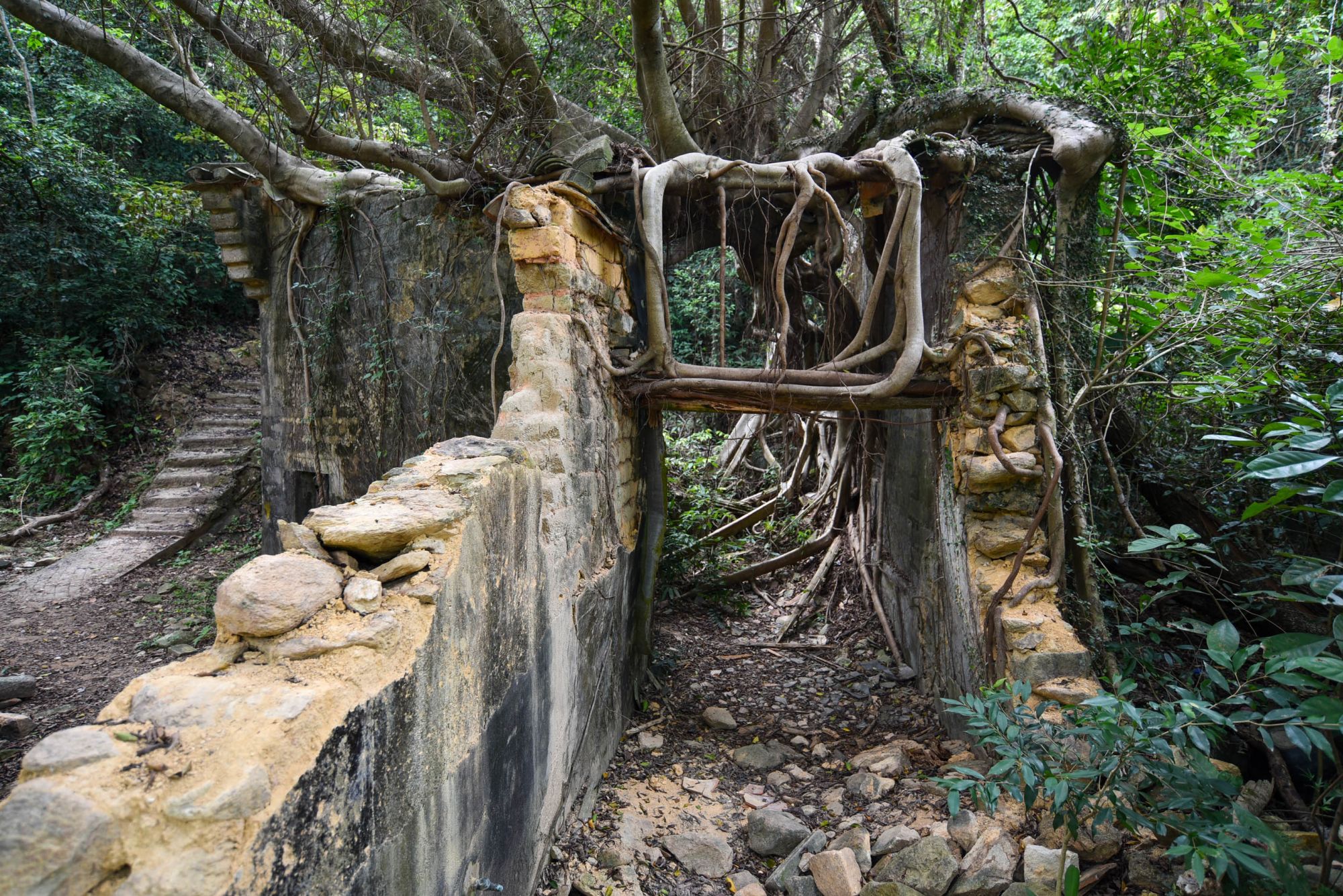The image depicts an outdoor scene set in a lush, forested area, rich with greenery, likely somewhere in Southeast Asia, possibly near Angkor Wat. The centerpiece of the photograph is a pair of ancient stone walls, light gray and white with dark patches, which have partially crumbled. Intriguingly, a network of tree roots has grown over and through the remaining structures, creating a natural roof-like formation connecting the walls. This organic growth includes both large roots and branches that envelop the scene, adding a mystical quality. The ground between the walls is a narrow, rocky pathway, covered with stones. To the left, a small set of stone steps leads up a gentle incline. The entire image is brightly illuminated by natural sunlight, enhancing the vivid greens of the trees, grass, and bushes, and the varied hues of the ancient stone and roots. This harmonious blend of decayed man-made architecture and robust natural elements highlights the passage of time and the intermingling of human history with nature.